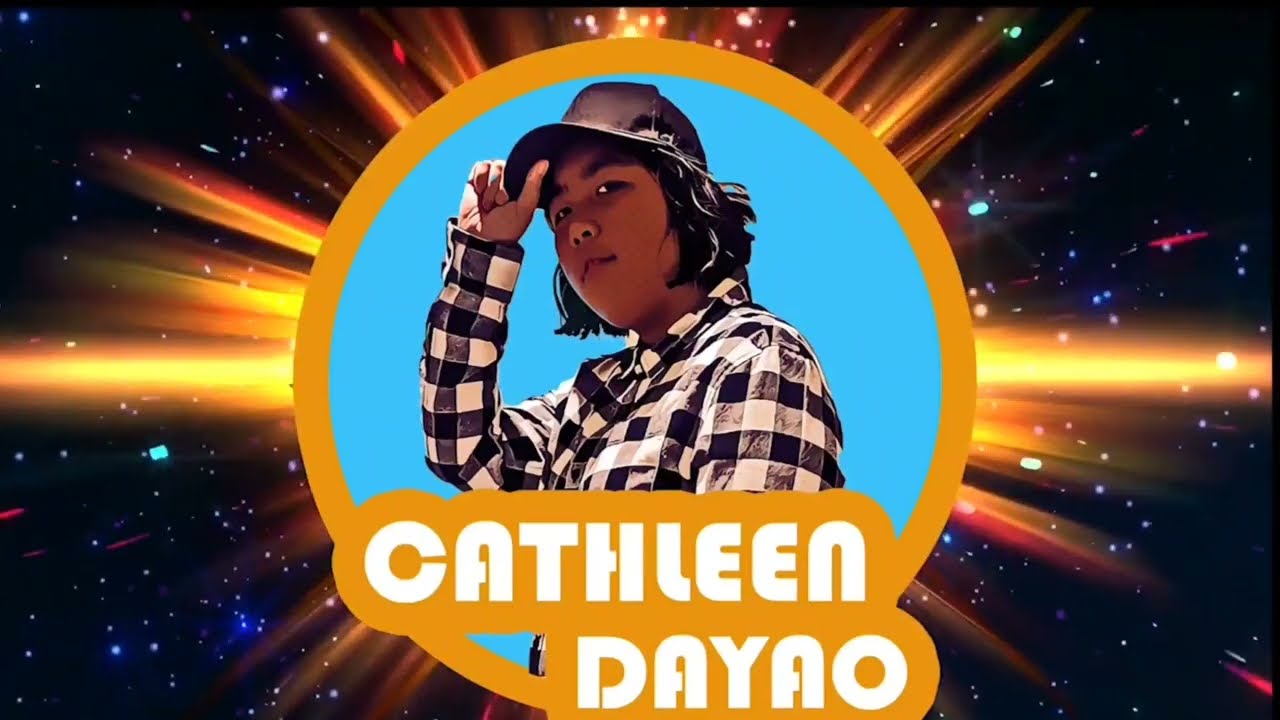The image showcases Kathleen Dayao, a young Chinese-Filipino woman from Manila, Philippines, who is a traveler, graphic designer, and vlogger. She is centrally positioned within an orange circle that takes up most of the graphic. This primary circle is surrounded by rays of yellow and orange, which resemble sunbursts extending outward to a star-studded, cosmic-looking background, reminiscent of images from the Hubble Space Telescope. Kathleen wears a black baseball cap, which she holds by the brim with her right hand. She is dressed in a black and white checkered long-sleeve flannel shirt, with her short hair ending just at her neck. Beneath her, in thick, uppercase white lettering with an orange border, is her name, "Kathleen Dayao." The blue background behind her adds a soft contrast to the vibrant orange circle and radiant cosmic rays.